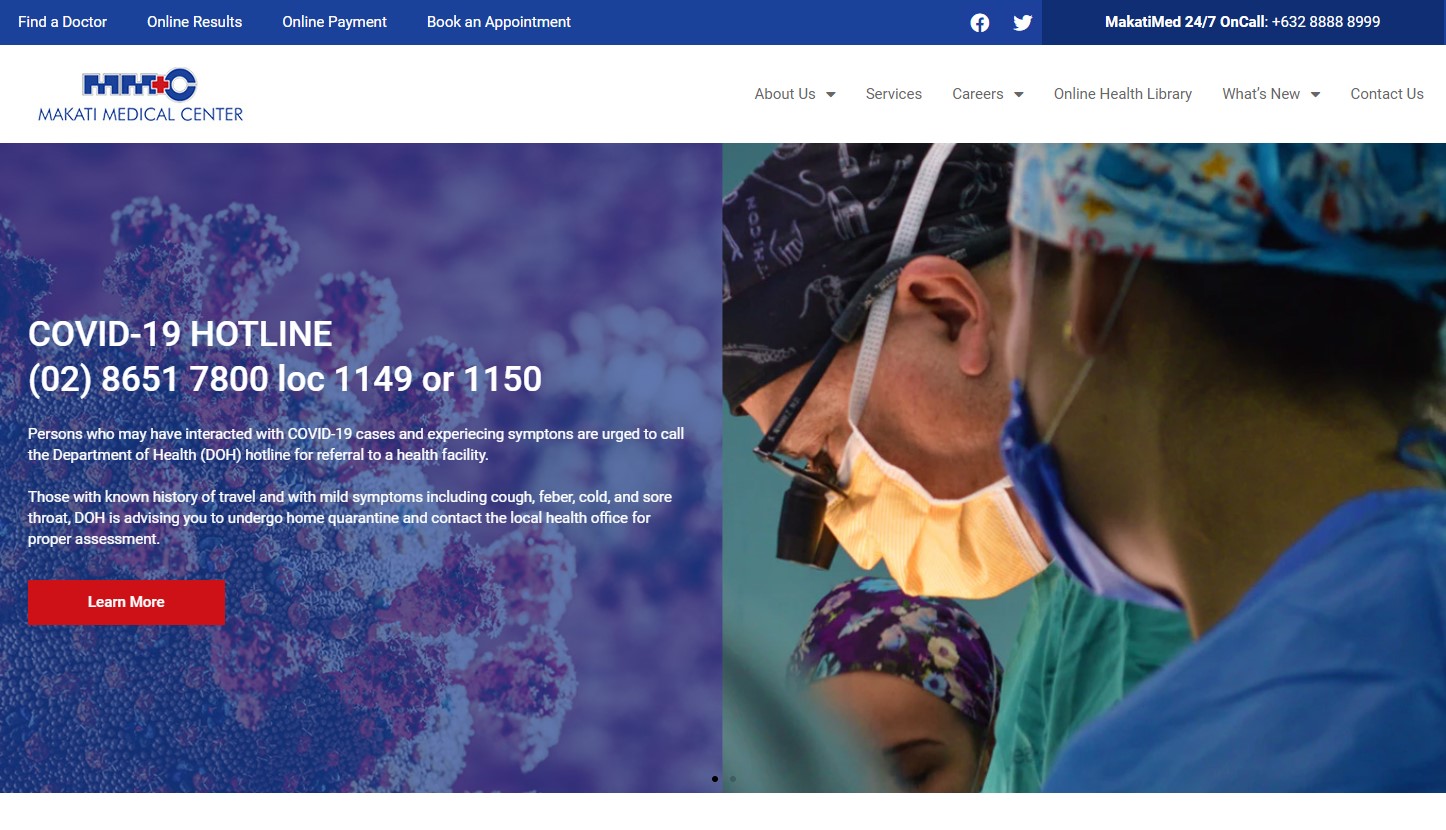The top section of the image features a blue rectangle with white text listing various online services: "Find a Doctor," "Online Results," "Online Payment," and "Book an Appointment," all aligned on the left-hand side. To the right, the image displays icons for Facebook and Twitter, accompanied by some indiscernible text and a sequence of numbers. Below these icons, there's a stylized text that reads "M+C," with the "M" in blue and the "+" in red, likely referencing the Makati Medical Center.

Moving to the right side of the image, there are several navigation options: "About Us," "Services," an unclear option, "Online Health Library," "What's New" with a downward arrow indicating a drop-down menu, and "Contact Us."

On the left side of the image, there is a purple square with a COVID-19 graphic and the text "COVID-19 Hotline." Beneath, it lists the contact number "02-8651-7800, LOC 1149 or 1150," with additional unreadable white text underneath. A red rectangle below this section reads "Learn More."

To the right-hand side of the image, there is a picture showcasing a doctor and several nurses, indicating the healthcare services provided.